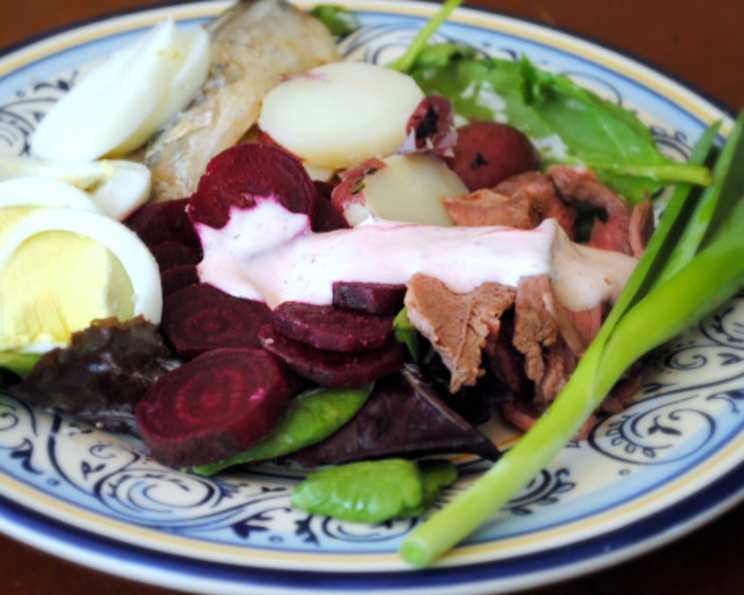The image showcases a beautifully presented salad on a fine blue china plate, which features a simple design of swirls and floral elements along the edges. The plate itself is white with dark blue and light blue accents, and it sits on a brown table. The vibrant salad includes sliced red beets, mixed greens of green and dark purple hues, sliced eggs, radish, boiled potatoes, and a scallion. Additionally, there appears to be some uncertain meat, possibly turkey or gyro lamb, drizzled with a white dressing that resembles ranch or tzatziki. The colors are striking, with the reddish-purple beets, green lettuce, white eggs, and the creamy dressing standing out prominently.